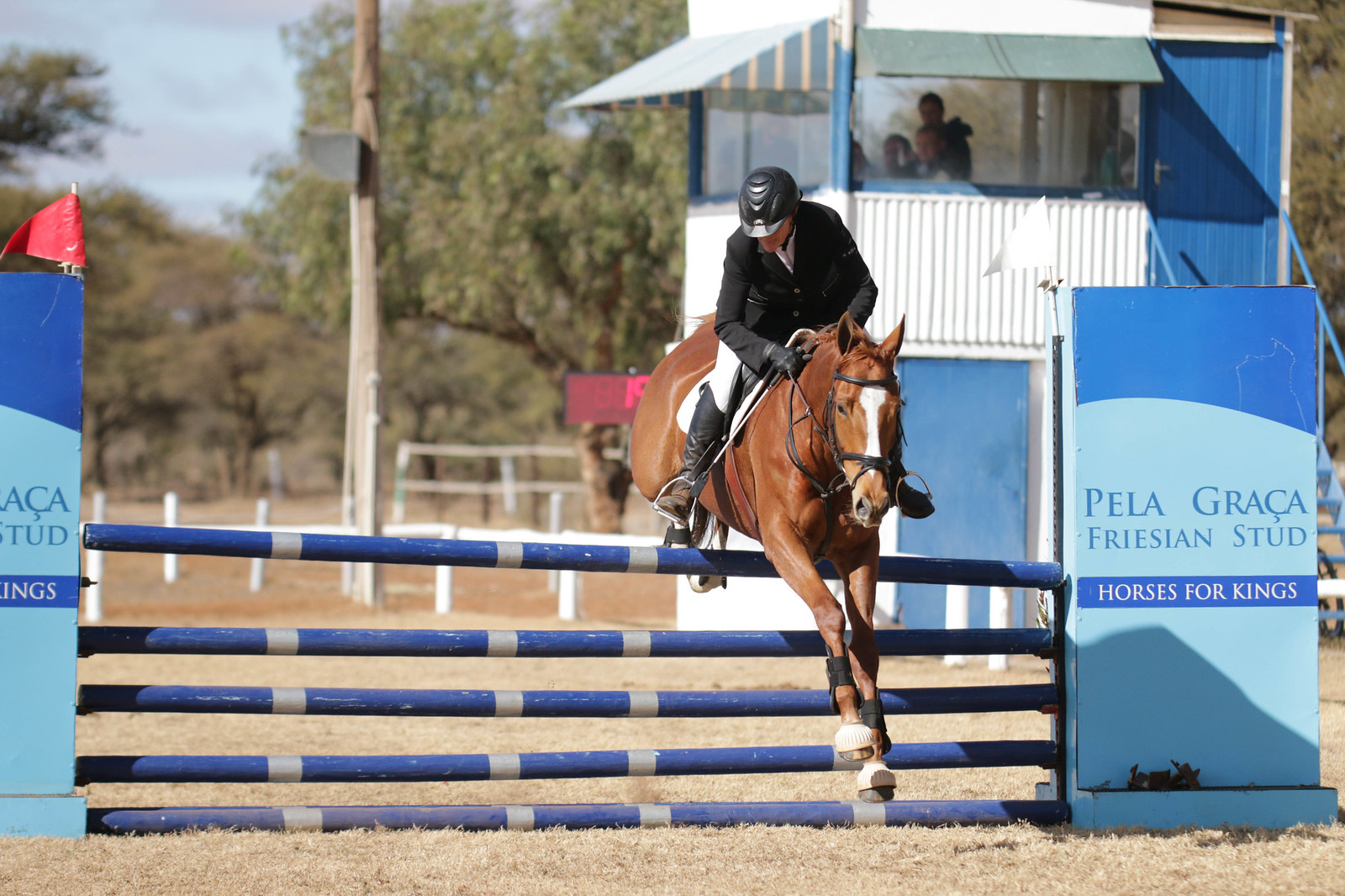The image depicts an equestrian sports competition set against a background of green trees and a blue sky. Central to the scene is a brown and white horse, captured mid-jump over a set of five blue and white striped wooden poles, about two to three feet high. Riding the horse is a person in a black jacket, black helmet, white pants, and black boots. Prominently displayed on both sides of the jump are signs, partially cut off, that read "Pellegrasse Friesian Stud Horses for Kings" in light and dark blue colors. Above these signs are flags, with a red flag to the left and a white flag to the right. In the backdrop, a white fence delineates the area, accompanied by a brown post extending out of the picture with a black box on top. To the far right, there stands a two-story structure with a blue and white striped awning and a second, darker blue awning. This structure serves as a viewing booth for spectators, several of whom are visible on the second floor.